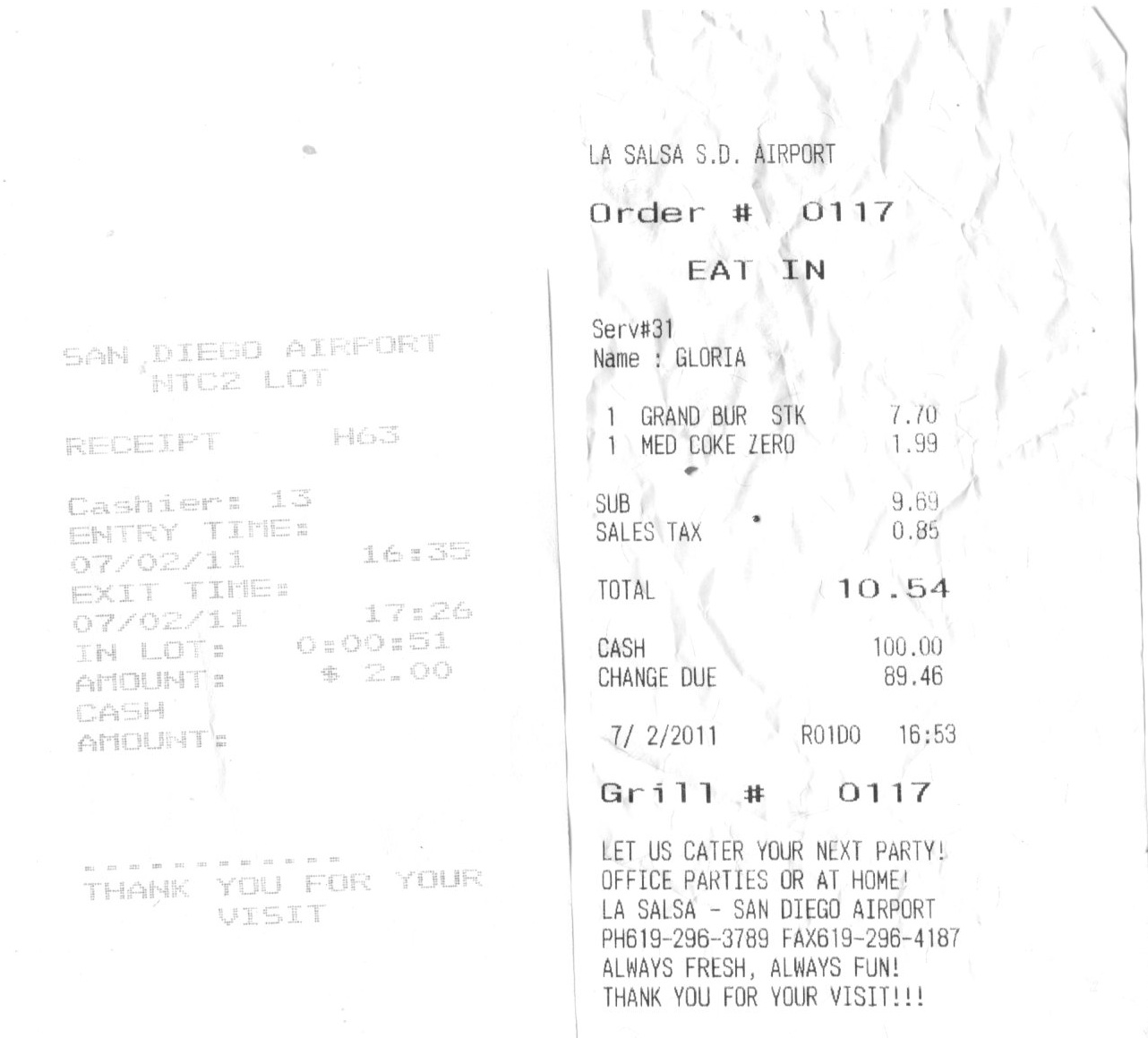The image features two detailed scans of receipts, likely associated with transactions at the San Diego Airport on the same date, 7/11. The first receipt, positioned on the left, is from "San Diego Airport NTC2 LOD" and is labeled as receipt H63, cashier 13. The parking entry time noted is 16:35, and the exit time is 17:26 on the same day. The total parking fee was $2. 

The second receipt, on the right, is from "LA Salsa SD Airport EN". The items purchased include a Grand Burger Steak priced at $7.70 and a medium Coke, priced at $1.99. The total amount for this transaction, including tax, is $10.54. Additionally, this receipt also mentions the date 7/11 and contains a promotional message at the bottom, encouraging customers to consider their catering services for their next party, accompanied by their contact information.